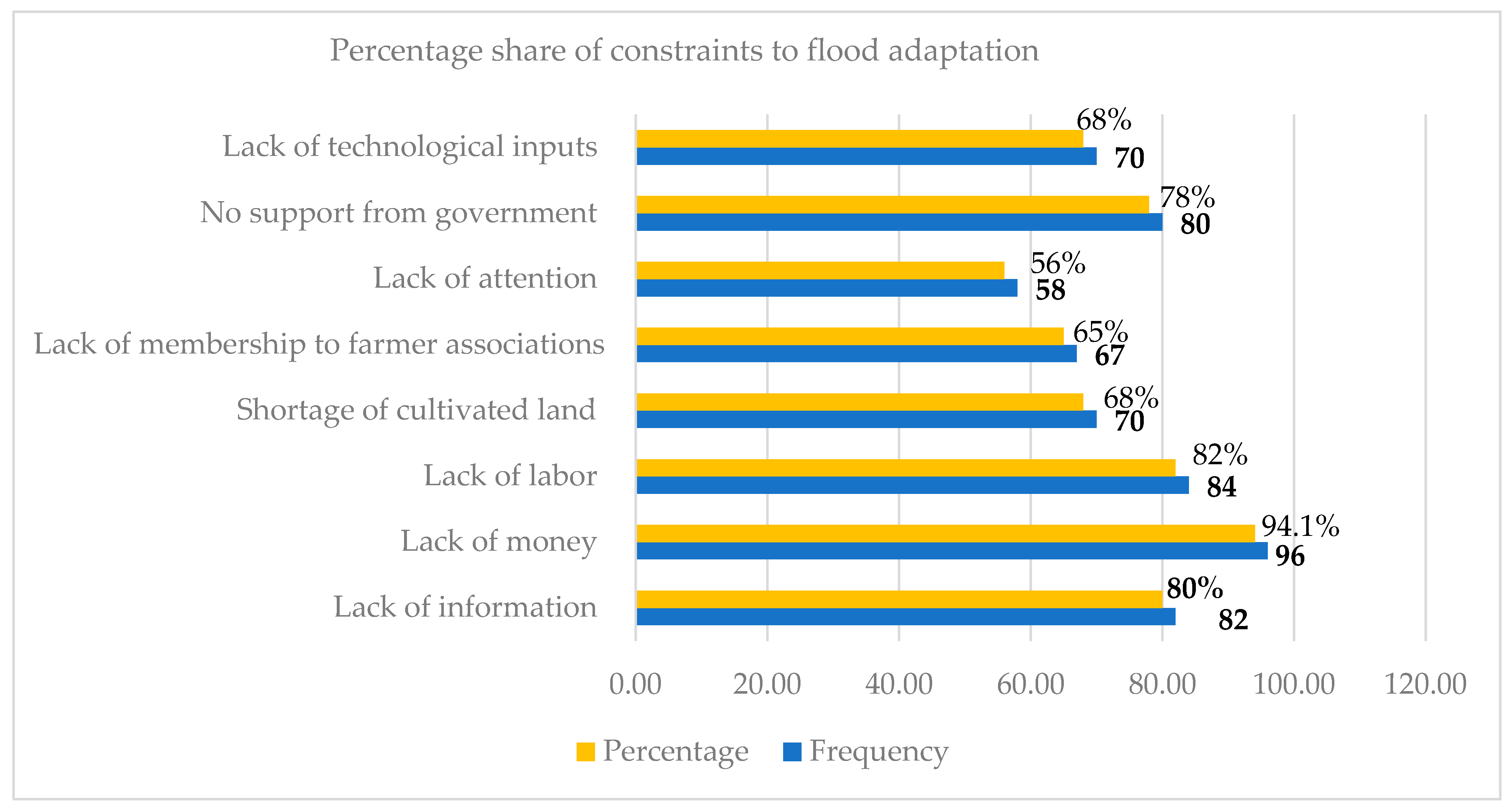The graph, encased in a thin gray border and wider than it is tall, is titled "Percentage Share of Constraints in Flood Adaptation." On the left side, various commodity-related issues are listed in rows from top to bottom: lack of technological inputs, no support from the government, lack of attention, lack of membership in farmer associations, shortage of cultivated land, lack of labor, lack of money, and lack of information. To the right of each listed issue, two lines—one yellow and one blue—represent percentages and frequencies, respectively. The yellow line (percentage) for "lack of technological inputs" reaches 68%, while the blue line (frequency) reaches 70%. The horizontal axis at the bottom of the chart is marked from 0 to 120 in increments of 20. It is noted that the yellow color represents percentage and blue represents frequency, with "lack of money" having the highest values in both categories.